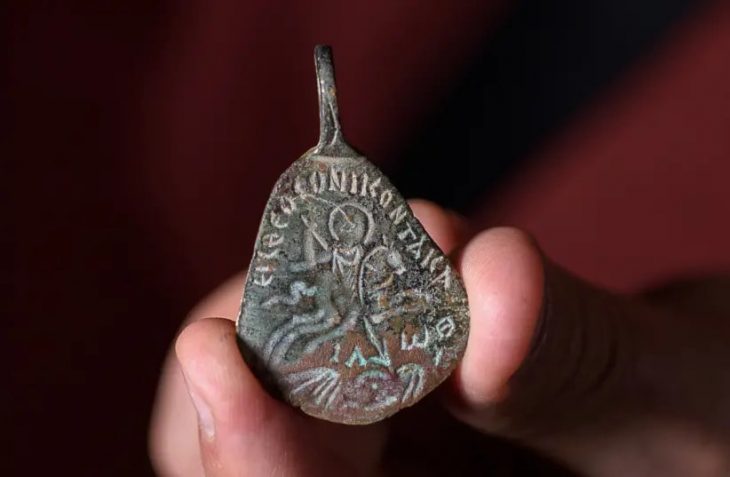In this detailed close-up photograph, one can see a hand holding a small, pear-shaped stone pendant. The background features a gradient of deep reddish tones interspersed with shadows, adding to the ancient and mystical feel of the scene. The hand, with visible fingers and white skin, delicately grasps the pendant with the thumb and three fingers.

The pendant itself appears to be an intricately hand-carved artifact, possibly made from a grayish stone with hints of green and red hues. It has a distinctive stem-like loop at the top, reminiscent of a fruit such as a pear or apple. The surface of the pendant features detailed carvings including what seems to be a simplified silhouette of a man, possibly a rider on a horse, and winged motifs with a circle between the wings at the bottom.

Along the top and bottom borders of the pendant, ancient-looking text is carved in white, partially legible with fragments resembling "E-L-E-F-O-U-N-I-K-O-N-T-A-K-A." The letters and figures suggest an artifact from a long-gone civilization, rich in history and emblematic of a bygone era.